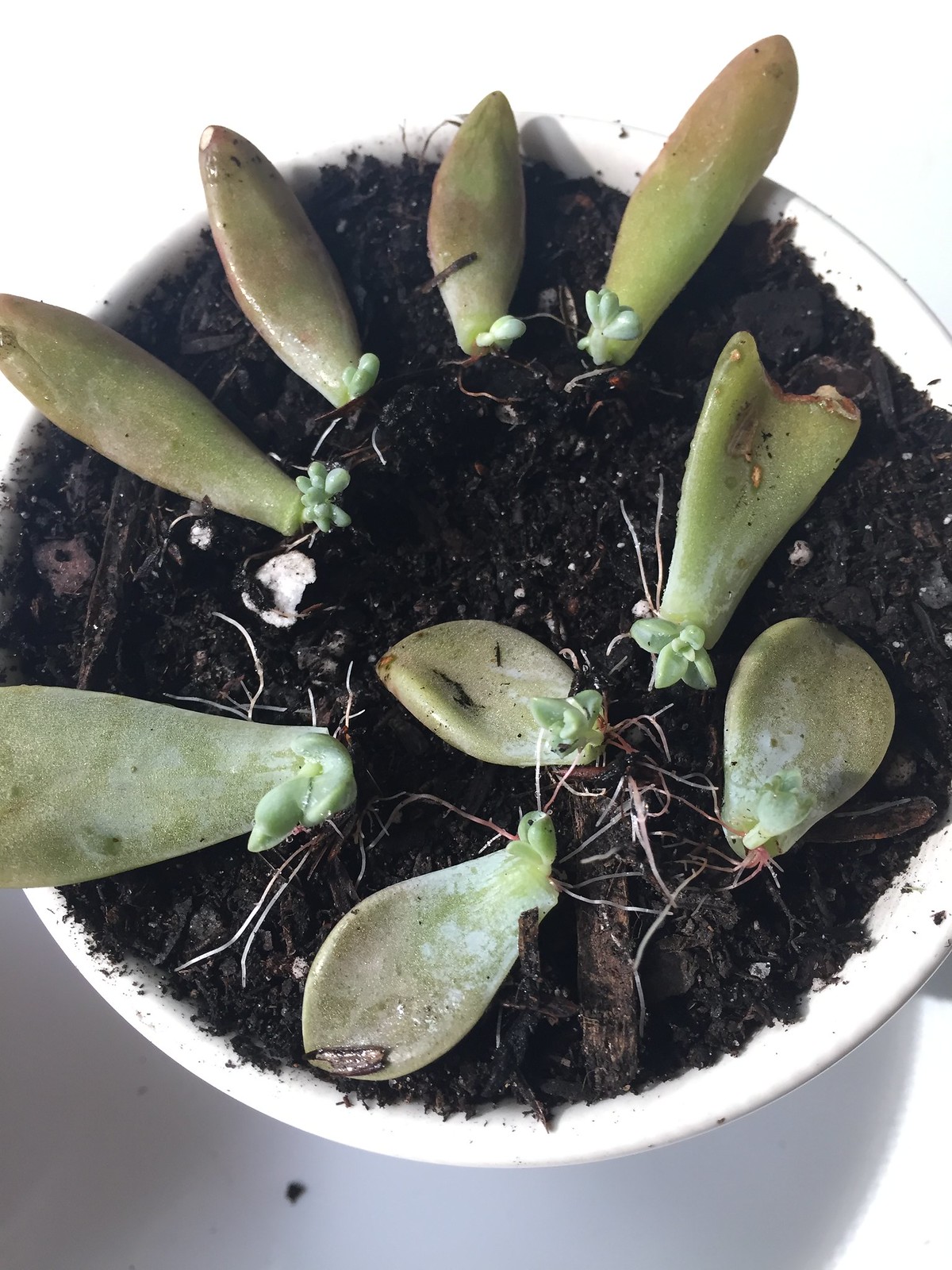The image showcases a close-up view of a white ceramic plant pot taken from above. The pot is filled with a rich, dark brown soil interspersed with lighter brown hues. Within the soil, delicate, paper-thin roots, resembling strands of hair, are visible and stretch across the left and right lower sides of the pot.

The main attraction is a cluster of small, succulent plants emerging from the soil. These plants, believed to be in the early stages of growth, have leaves varying slightly in shape and size. Most leaves are teardrop-shaped or flat at the end and possess a rubbery consistency typical of succulents. They exhibit a light green color, transitioning to even brighter green at the tiny offshoots or baby leaves sprouting from their ends.

The succulent leaves are nearly the length of a quarter, with some just as wide while others are thinner. These puffy, circular leaves, some bean-like at their tips, appear similar to aloe leaves, though they are smaller and in the propagation phase. The fine, white and light gray roots at the base of these leaves are beginning to establish, indicative of a meticulous propagation process where they are misted regularly to encourage further growth.